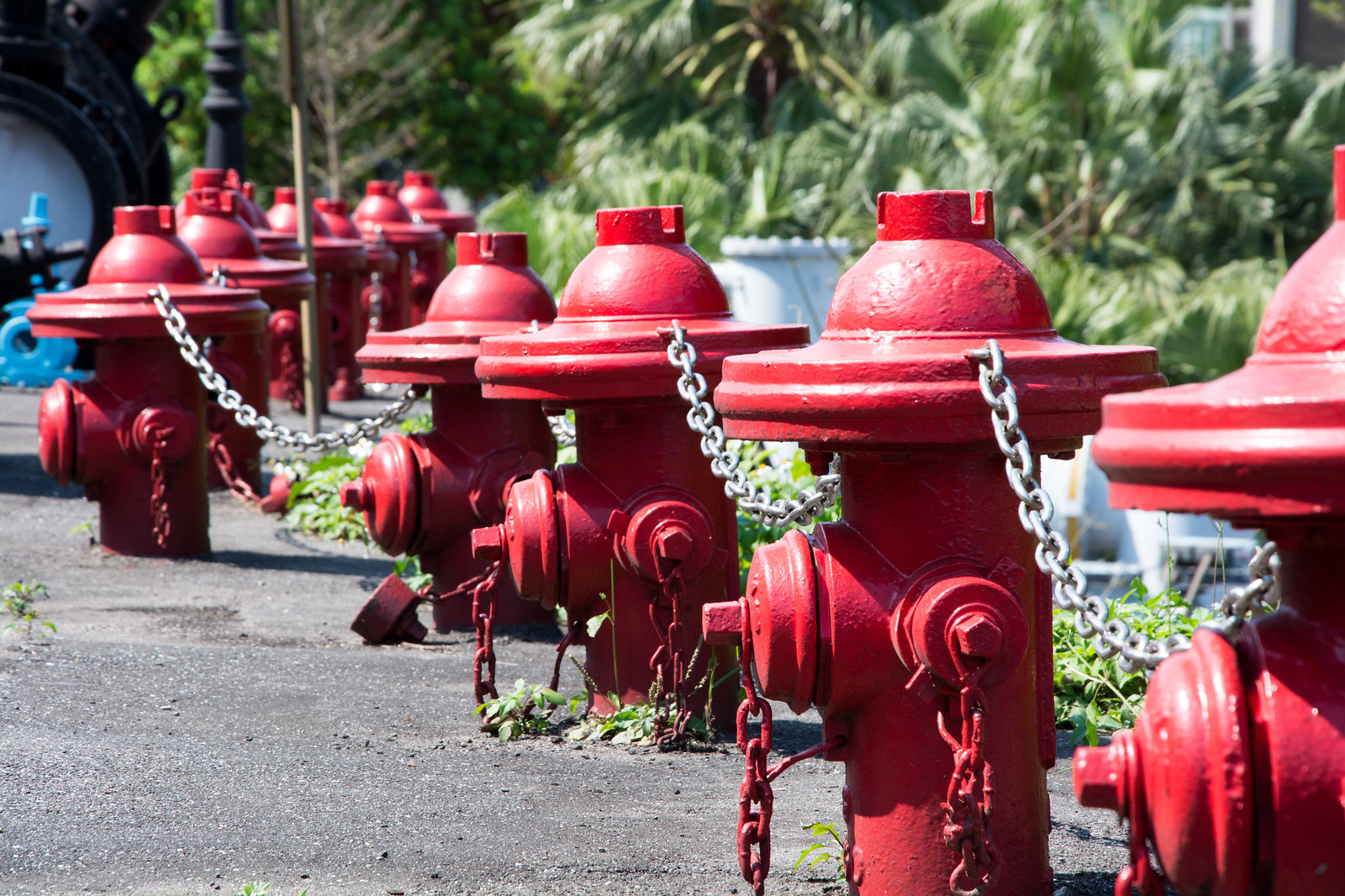The image depicts a slightly wider-than-tall outdoor scene with a gray cement road curving from the lower right-hand corner to the center left, then veering off to the right. Lined up in a neat row along the edge of this road are approximately 11 to 15 old-fashioned red fire hydrants, each linked by a heavy silver chain connected to the hydrants' top outer lids. Additional red chains hang from the bolts on the front and side of each hydrant, connecting their spigots. The road appears to be on the right side, while the left features some light gray pavement. 

In the background, lush green trees and grass-like vegetation provide a verdant backdrop, interspersed with various elements like a bare tree and a tall palm tree with a brown trunk. There are also several structures and objects: a tall black or dark green street lamp, a black circular object, a blue water device-like object, and an obscured sign. These hydrants, set against the greenery, possibly create a decorative fencing effect to delineate or mark off an area.